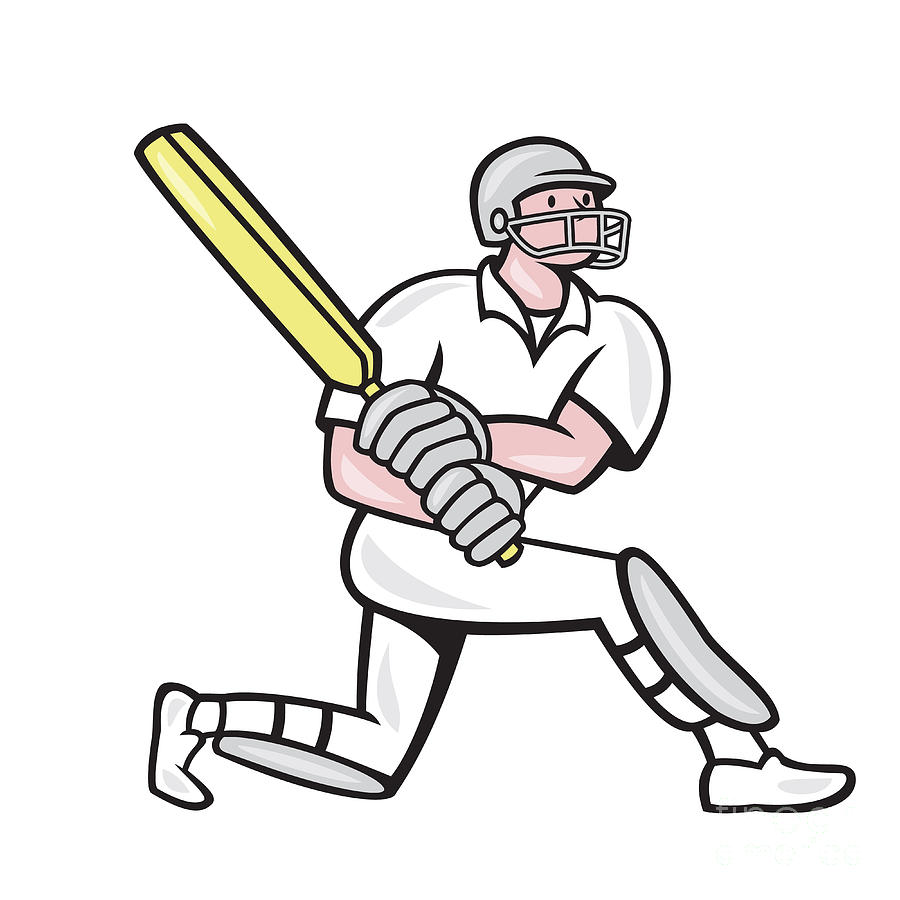This detailed cartoon drawing depicts a cricket player captured in mid-swing, likely having just connected with a pitch. The illustration, with its black outlines and simple color palette, shows the player with pink skin, black eyes, and a light pink face. He is dressed in a white uniform consisting of a shirt and pants, complemented by gray shin pads and heavily padded gloves. The player also sports white slip-on shoes and a gray helmet with a face mask for protection. His yellow cricket bat is held high, indicating an aggressive stance towards the low pitch he's poised to strike. One of his knees is bent and touching the ground, while the other leg is extended with the foot flat on the ground, reflecting the classic posture of a cricket player at the moment of the swing. The entire figure has a slightly caricatured style, suggesting it could be either a hand drawing or created with computer software.